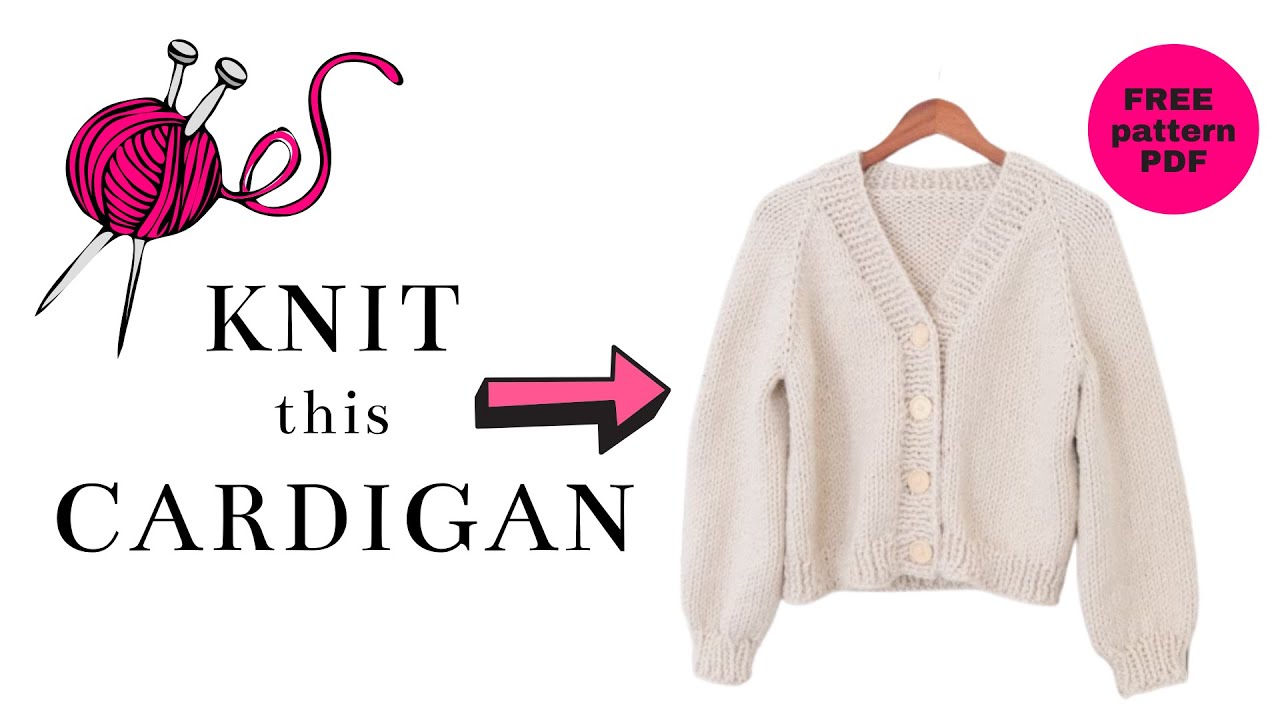The promotional image features a clean, rectangular white background, with the top and bottom edges twice as long as the left and right edges. In the top right corner, a neon pink circle contains the black text "Free Pattern PDF" in a sans serif font. Below and slightly to the left of the circle, a knit sweater is displayed, buttoned up with large white buttons and hanging from a wooden clothes hanger. To the left of the sweater, black serif text reads "Knit this Cardigan," accompanied by a pink arrow with a black border pointing towards the sweater. In the top left corner, a cartoon graphic of pink yarn with two large silver knitting needles piercing through it adds a whimsical touch to the design. This image clearly communicates that it is promoting a free knitting pattern for the displayed cardigan.